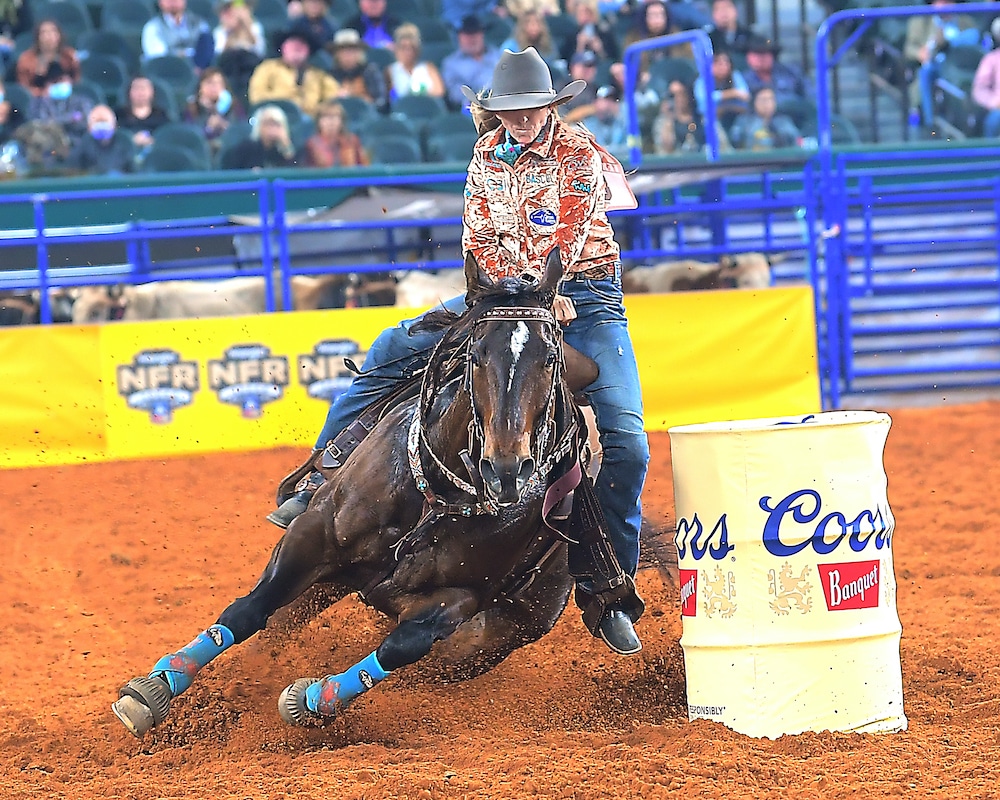In this dynamic image taken at a rodeo competition, a female rider skillfully maneuvers her powerful, dark brown horse around a Coors Banquet barrel, tilted at a dramatic 45-degree angle. The horse, sporting blue leg wraps and a distinctive white patch on its forehead, has its legs splayed to balance the high-speed turn, showcasing its agility and strength. The rider, with remarkable poise, remains completely perpendicular to the ground, dressed in a distinctive grey cowboy hat and a vibrant red, white, and possibly yellow patterned shirt adorned with sponsor labels. She complements her outfit with light blue jeans and black boots. Surrounding the action, the scene is set on brownish-red dirt and framed by blue railings and a yellow banner. In the background, blurred spectators and penned livestock add to the authentic rodeo atmosphere.